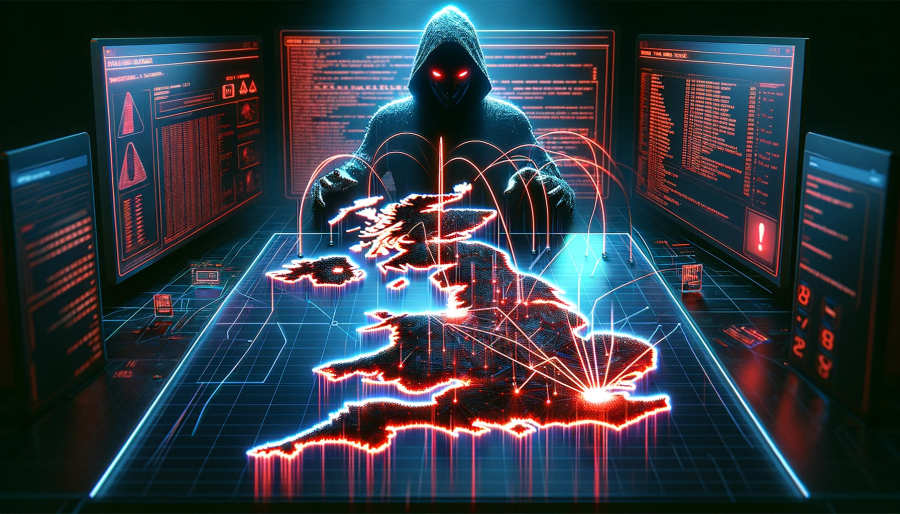In this AI-generated digital illustration, a menacing demon-like figure shrouded in a dark, hooded cloak with red glowing eyes stands ominously behind a futuristic, holographic table. The rectangular table emits a blue light and features a grid with a detailed, 3D map that resembles land areas but not any specific real-world location. This map is animated with orange, flame-like electric electrodes popping out sporadically, and red lines that appear to denote connections or missile trajectories, evoking a scene from a futuristic war game. The figure's clawed hands are raised as if orchestrating chaos on the map. Surrounding this sinister character are multiple computer screens, lit up with orange and red digital codes, words, and letters, enhancing the dark and ominous cyber hacker atmosphere.